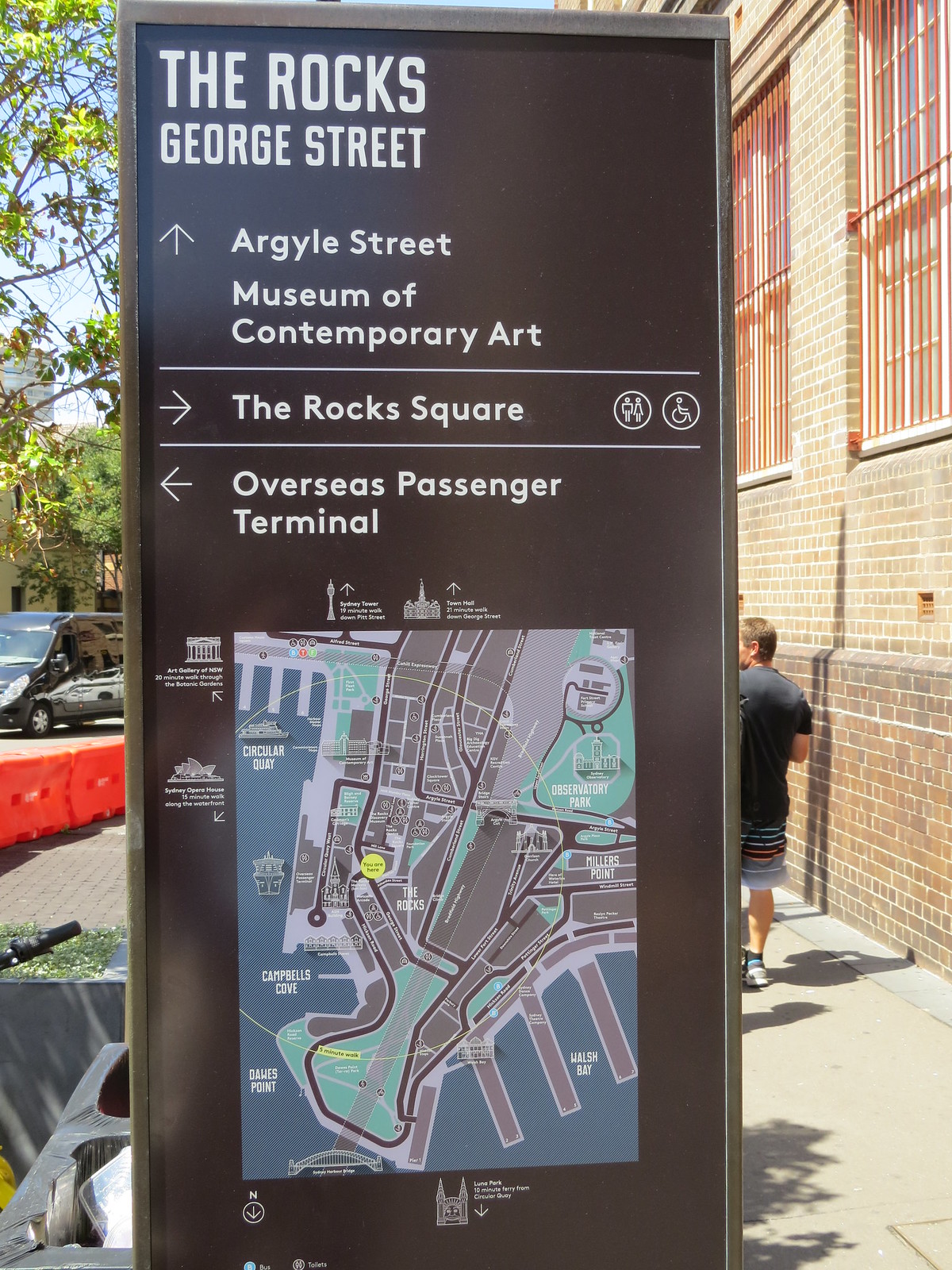This photograph captures a detailed street scene in a city, centering on a large, prominent street sign. The sign, primarily a map, occupies about half of its total area. It is color-coded in shades of pink, light blue, and dark bluish-gray, with well-labeled streets and notable landmarks. The map includes a yellow dot for reference points and displays "The Rocks, George Street" at the top. Arrows on the sign direct viewers to various points of interest: an upward arrow points to Argyle Street and the Museum of Contemporary Art, a rightward arrow indicates The Rock Square, and a leftward arrow guides toward the Overseas Passenger Terminal. Additionally, the map highlights locations such as The Rocks, Observatory Park, Circular Quay, and Campbell's Cove.

In the foreground, a man in a blue shirt and shorts is walking away from the camera on the sidewalk, his face not visible but his shadow clearly cast on the ground. Surrounding elements include a brick building on the right, a street to the left, a van in the background, and orange traffic barriers, contributing to the urban atmosphere.